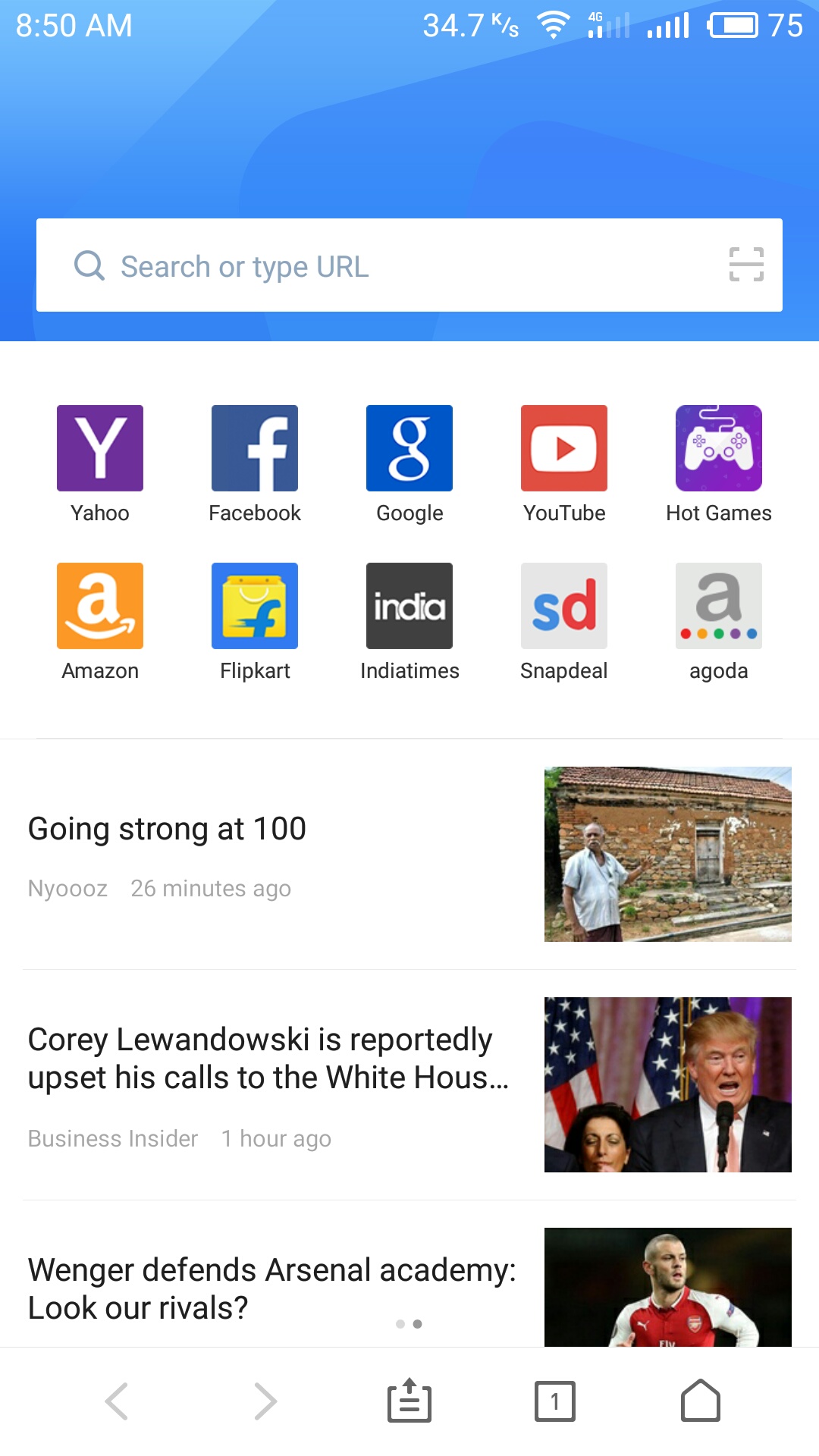**Caption:**

This screenshot displays a phone interface featuring a search bar at the top labeled "Type search or type URL." Below the search bar are two rows of five app icons each with their respective names in dark grey text. The apps include Yahoo, Facebook, Google, YouTube, and Hot Games.

Beneath the apps is a list of three news stories:
1. **"Going Strong at 100"**: The image accompanying this story shows an elderly man wearing a shirt, standing in front of a dilapidated brick cottage with no windows. He is pointing towards the cottage.
2. **"Corey Lewandowski is Reportedly Upset"**: This story features a photograph of Donald Trump speaking at a microphone with American flags draped behind him, and a staffer standing in the background.
3. **"Wenger Defends Arsenal Academy: Look at Our Rivals"**: Accompanying this headline is an image of a footballer running on the field.